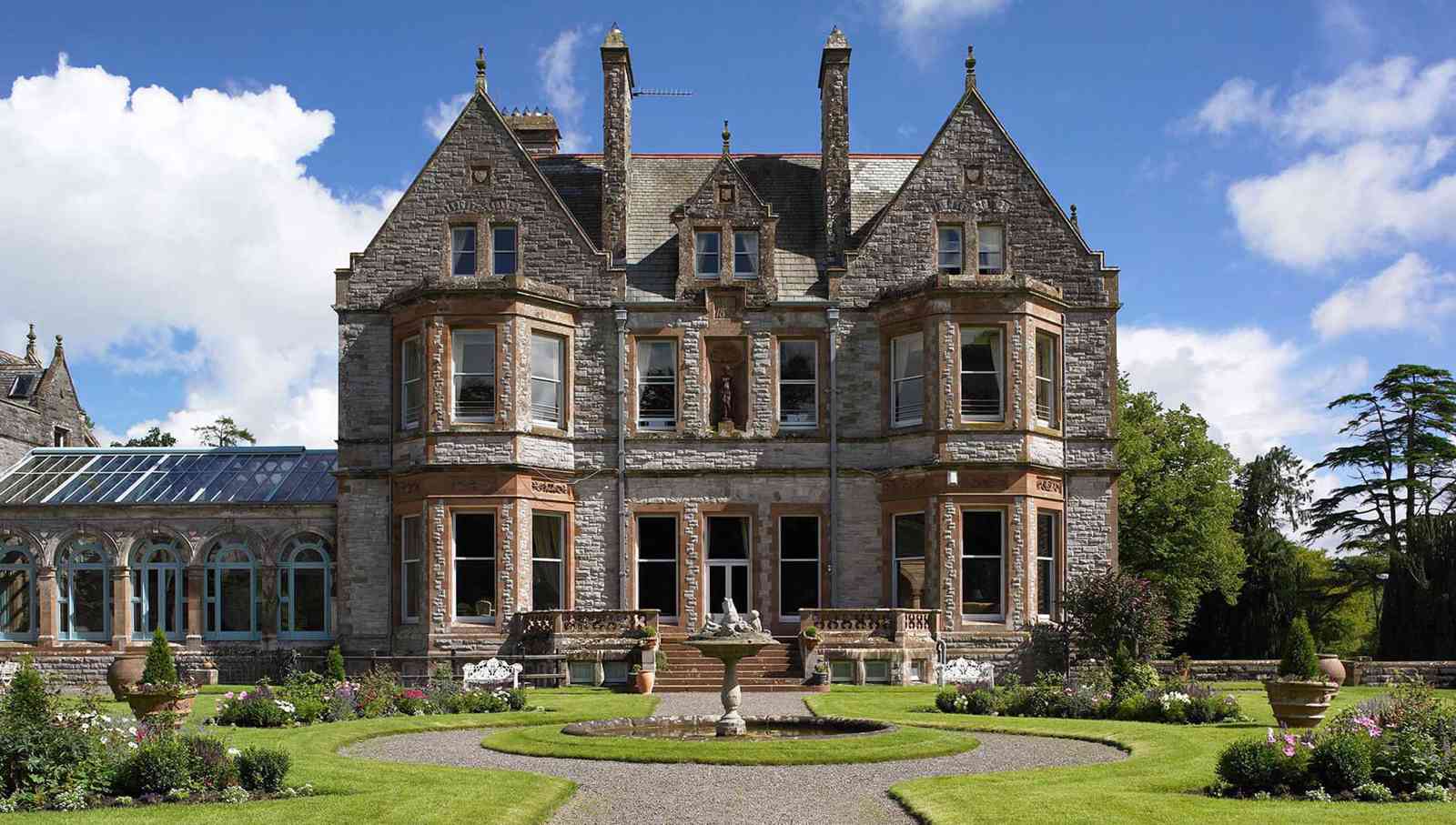This photograph showcases a grand, castle-like mansion known as Castle Leslie, observed in exquisite detail. The mansion, constructed with a blend of beige and gray stone and adorned with striking orange trim around the windows, stands prominently in a lush, well-manicured garden. The house rises to three stories, with two main levels crowned by an attic area. The front facade features steep awnings, two grand spires, and two ornate chimneys. 

At the entrance, an imposing stone stairway leads up to double doors, flanked by smooth, brown cement pillars and decorative stone railings. At the heart of the circular driveway in front of the house lies a marble fountain, encircled by a graveled path. Bordering the walkway are vibrant flower beds with red, pink, and white blooms, large potted plants, and white benches with detailed embroidery.

To the left of the mansion, there is a one-story greenhouse or solarium with large windows and a glass roof, seamlessly attached to the main structure. Flanking the building is a beautifully landscaped grassy lawn, dotted with small plants and large trees, which also populate the background against a bright blue sky filled with puffy white clouds.

Overall, Castle Leslie presents a harmonious blend of architectural grandeur and meticulous gardening, framed by a serene, sunny day.